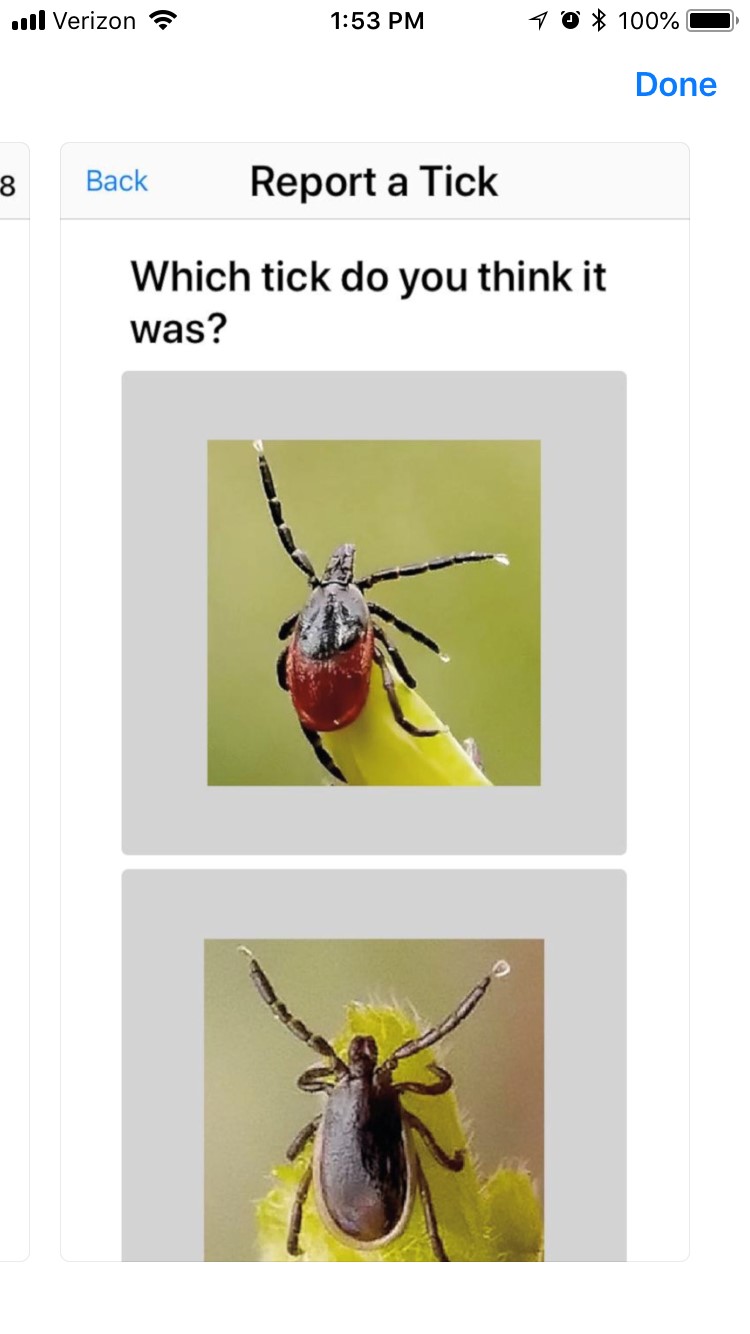The image is a detailed screenshot from a mobile device displaying a report interface for identifying ticks. At the top, a gray banner reads "Back" in blue highlighted text. Below this banner, bold black letters state, "Report a Tick," followed by the question, "Which Tick Do You Think It Was?" on a white background. Beneath the text are two framed images of different ticks. The first tick, positioned on a yellow-green leaf, shows a multicolored body with a reddish-brown lower section and a black upper section, including black legs tipped with white. The second image depicts a more bulbous, all-brown tick with legs also tipped with white, resting on a similarly colored yellow-green plant with a fuzzy texture, against a blurred green background. The device status bar at the top of the image shows it is 1:53 PM, with icons for Verizon network signal, Wi-Fi, battery status at 100%, and other common notifications. On the upper right, the word "Done" appears in blue text.